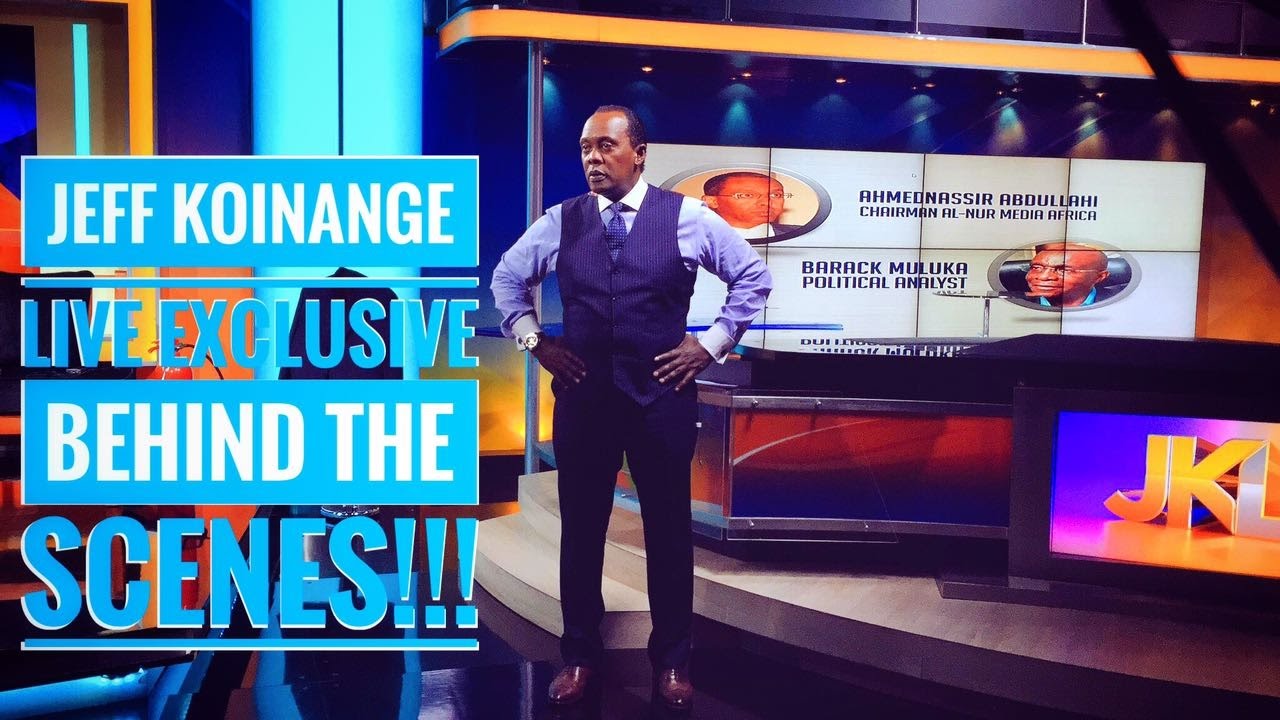The image is a detailed screenshot from a television show, likely set in a newsroom or production stage, featuring an exclusive behind-the-scenes segment with Jeff Coynage. In the center stands Jeff Coynage, a black man dressed in a dark purple vest over a light purple dress shirt, complemented by a dark purple tie, black slacks, and brown dress shoes. His attire is meticulously described, down to the vest's buttons and white collar.

On the left side of the image, prominent text reads "Jeff Coynage Live Exclusive Behind the Scenes." The words "Jeff Coynage" and "Behind the Scenes" are displayed in white text inside blue boxes, whereas "Live Exclusive" and "Scenes" appear in blue text with a subtle white drop shadow.

In the background, a large screen composed of smaller screens showcases two people inside circular frames with captions identifying them as Ahmed Sir Abdullahi, Chairman Al-Nur Media Africa, and Barak Moolaguluka, Political Analyst. Another digital screen prominently displays the initials "JKL" in large gold letters. The stage is well-lit with an array of digital signs, neon blue and yellow lights, and metal columns holding up a yellow balcony, further enhancing the newsroom ambience. The floor of the auditorium stage looks wooden, adding a polished touch to the setting.